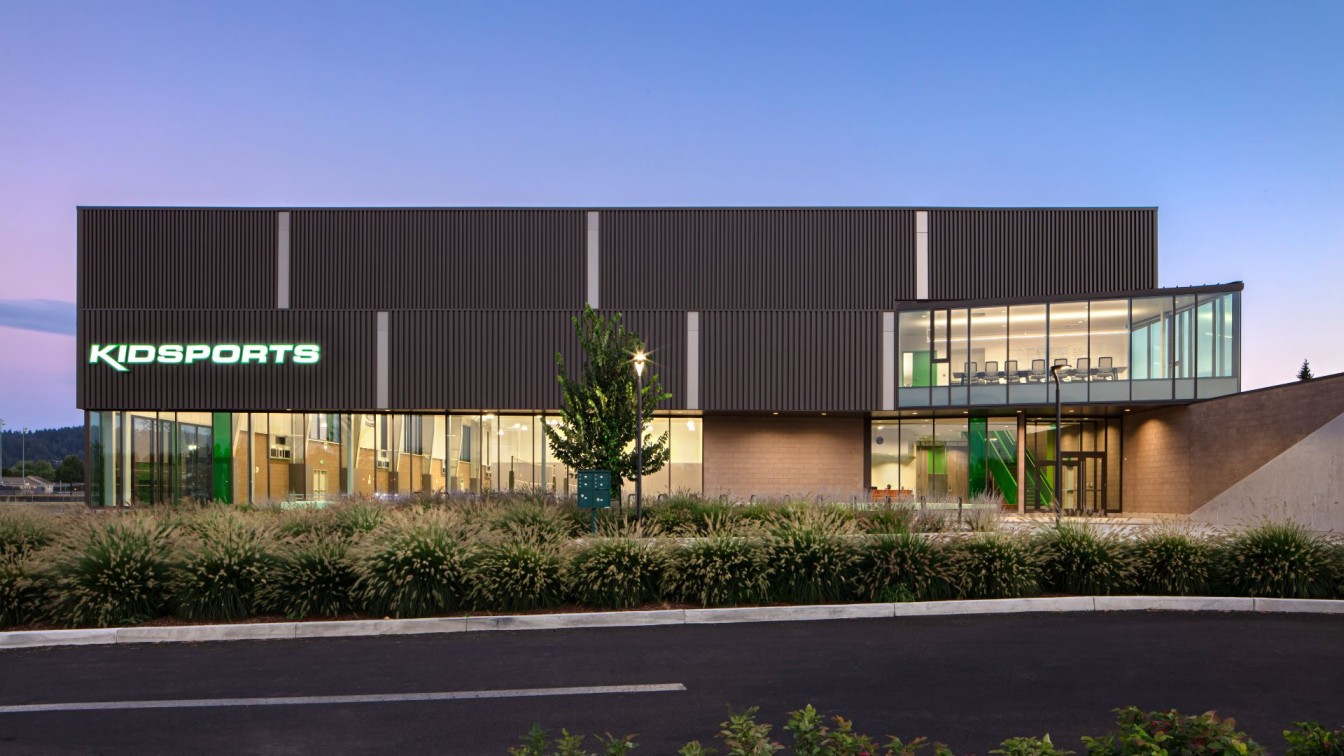The image depicts a modern, dark gray commercial building facing a divided roadway. The building features three distinct levels. The ground level, comprised of glass siding, showcases a brick base and an entrance with doors. There are windows along this level allowing a glimpse into the interior, including chairs and other furnishings. Above it, the second level is also lined with glass, revealing a large meeting room with a big table and numerous chairs. 

The building is adorned with vertical black lines and gray pipes running down its exterior. A lit sign displaying "Kids Sports" in white letters is prominently positioned on the bottom part of the roof, marked by three gray lines. Surrounding the building's perimeter are lush green and white bushes and a small tree, contributing to the landscaped appearance of the roadway. The evening sky in the background is a blend of purplish-blue hues with scattered clouds, adding a serene ambiance to the scene.